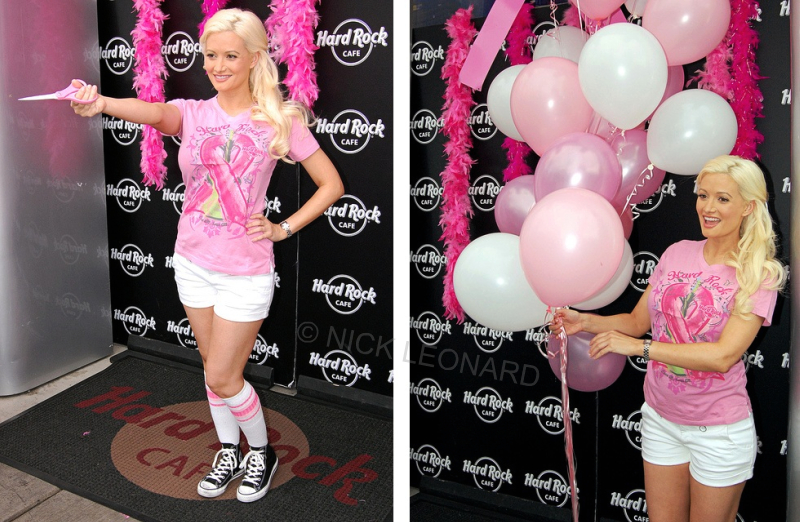The image comprises two photographs of Holly Madison, placed side-by-side, taken moments apart at the Hard Rock Cafe. In both photos, Holly stands before a black wall adorned with the Hard Rock Cafe logo and pink fuzzy boas. She is dressed in a pink cancer awareness t-shirt, white shorts, white socks with pink stripes, and white and black tennis shoes. Her blonde hair flows over her left shoulder. In the first photo on the left, Holly strikes a confident pose with her left hand on her hip and her right hand holding out a pair of pink scissors, suggesting she is about to participate in a ribbon-cutting ceremony. In the second photo on the right, she holds a cluster of pink balloons of varying shades, adding a celebratory atmosphere to the scene.